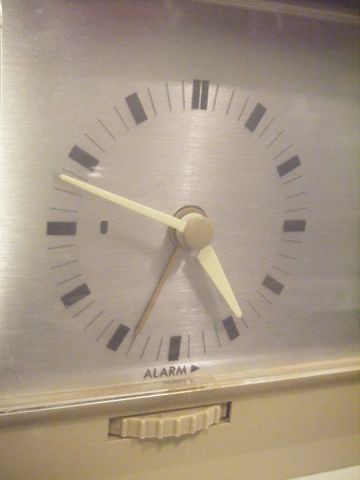This is an extremely detailed close-up photo of a modern alarm clock face. The clock, set against a stainless steel background, features a clean, eggshell white face devoid of traditional numbers. Instead, it uses bold black blocks to mark the hours, with the 12 o'clock position distinguished by two thin, elongated black rectangles. Between these blocks, smaller, thinner lines mark the minute intervals. The clock shows the time as approximately 10:10:30, with white hour and minute hands, and a thin seconds hand in a grayish beige color. Below the center of the clock face, the word "alarm" is clearly visible. Additionally, a small, yellowish plastic scroll button for setting the alarm is situated beneath the face. The image captures light reflections, emphasizing the metallic and slightly reflective nature of the clock's surface.